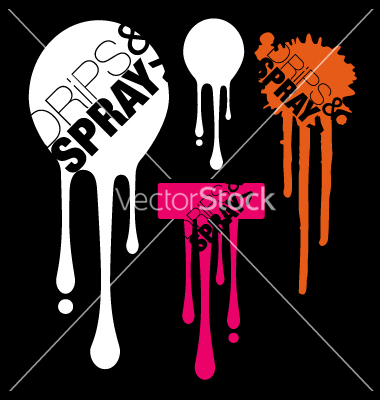In this striking and visually captivating image, we see a poster that exudes an edgy, graffiti-like aesthetic. The poster is square-shaped with a stark black background. A thin, white, diagonal X intersects the entire frame, giving the appearance of an envelope. The main focal points are four splattered paint shapes that seemingly drip down the canvas. 

On the left, a large white splat drips downward, with the words "Drips and Spray" written diagonally in black block letters. Opposite, to the right, is a smaller white shape, mirroring the larger one. Below these, centrally positioned, is a red splat with horizontal drips, while to its right lies a yellow splatter of paint. These vibrant spots and the dynamic drips create an array of movement across the composition. 

At the center of the canvas lies a watermark in white text reading "Vector Stock," suggesting this image is sourced from a stock illustration repository. The scattered yet deliberate arrangement of the colors—white, red, and yellow—stand out against the dark background, enhancing the poster's potential as an eye-catching advertisement, likely for a paint or spray paint product marketed in a store or home improvement setting.